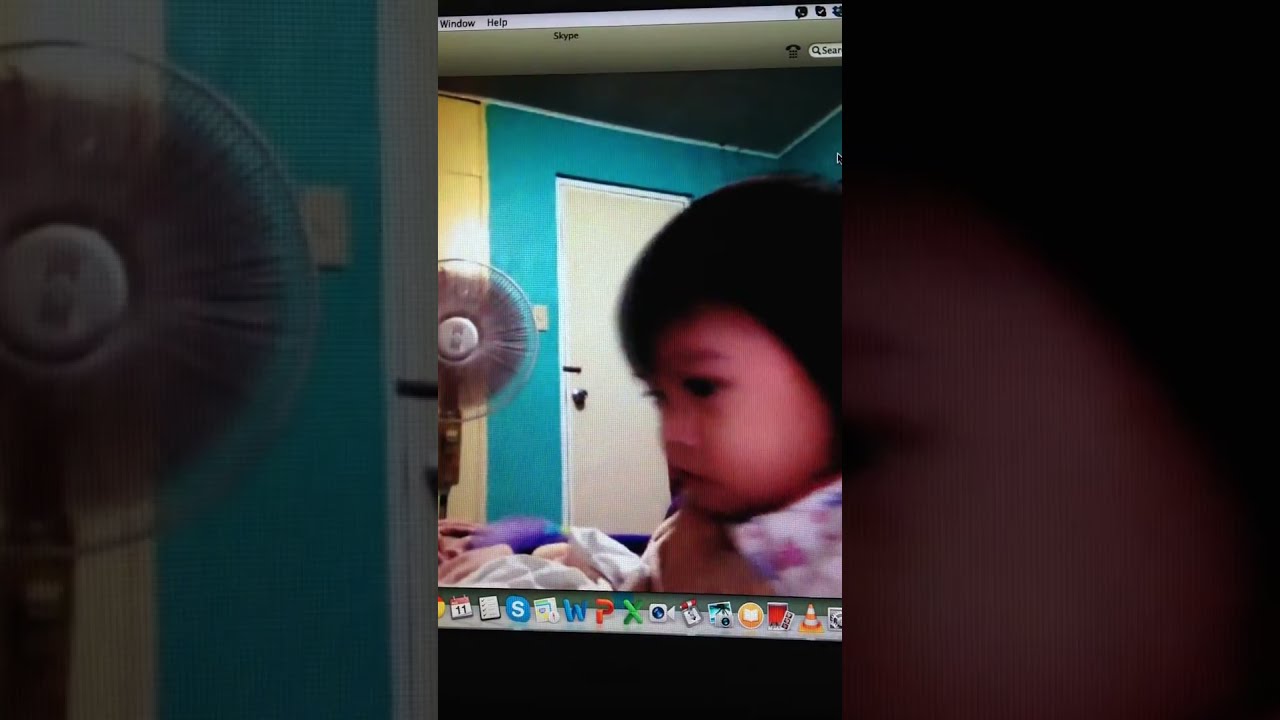This image is a photograph of a computer screen displaying a low-quality picture of a room, framed by thick, solid black borders on both the left and right sides. The picture reveals a room with turquoise blue walls and a white door, possibly beige with a white frame. The door, situated at an upward angle as if the photo was taken from the ground or a bed, dominates the center. To the left of the image, there's a circular floor fan in motion, appearing as a black-gray blur. Directly behind the fan, there's a yellow element, which could be part of the wall or a shelf. The right side features stacked items, suggesting a desk or shelving unit, though details are vague due to the poor focus and lighting of the photo. At the very bottom, a white blanket or sheet, possibly patterned with tan and hot pink, can be seen blurred in the foreground. The photograph is captured from a computer screen, as evidenced by the presence of a taskbar at the bottom showcasing various app icons such as a calendar with the number 11, Skype, a blue 'W' (likely Microsoft Word), a red 'P' (PowerPoint), a green 'X' (Excel), a camera, a safety cone (possibly VLC media player), and other icons, along with a mouse cursor near the top right corner.